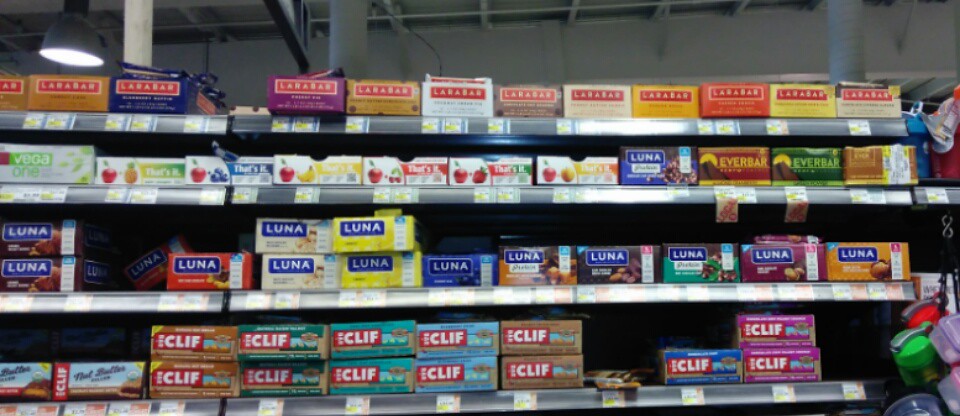In this photograph, the neatly organized shelves of a store display a diverse selection of granola bars and snacks. The image captures four shelves stacked with various brands and flavors. On the lowest shelf, an array of Clif bars is showcased, offering a variety to choose from. Above them, Luna bars make up the entire second shelf, followed by a collection of That's It snacks and another set of Luna bars on the third shelf. The top shelf features an assortment of Laura bars, all neatly lined up. Each product has an accompanying price tag, though they are too distant to discern the actual prices. The background reveals a plain white wall and an industrial-style ceiling, setting a typical store ambiance.